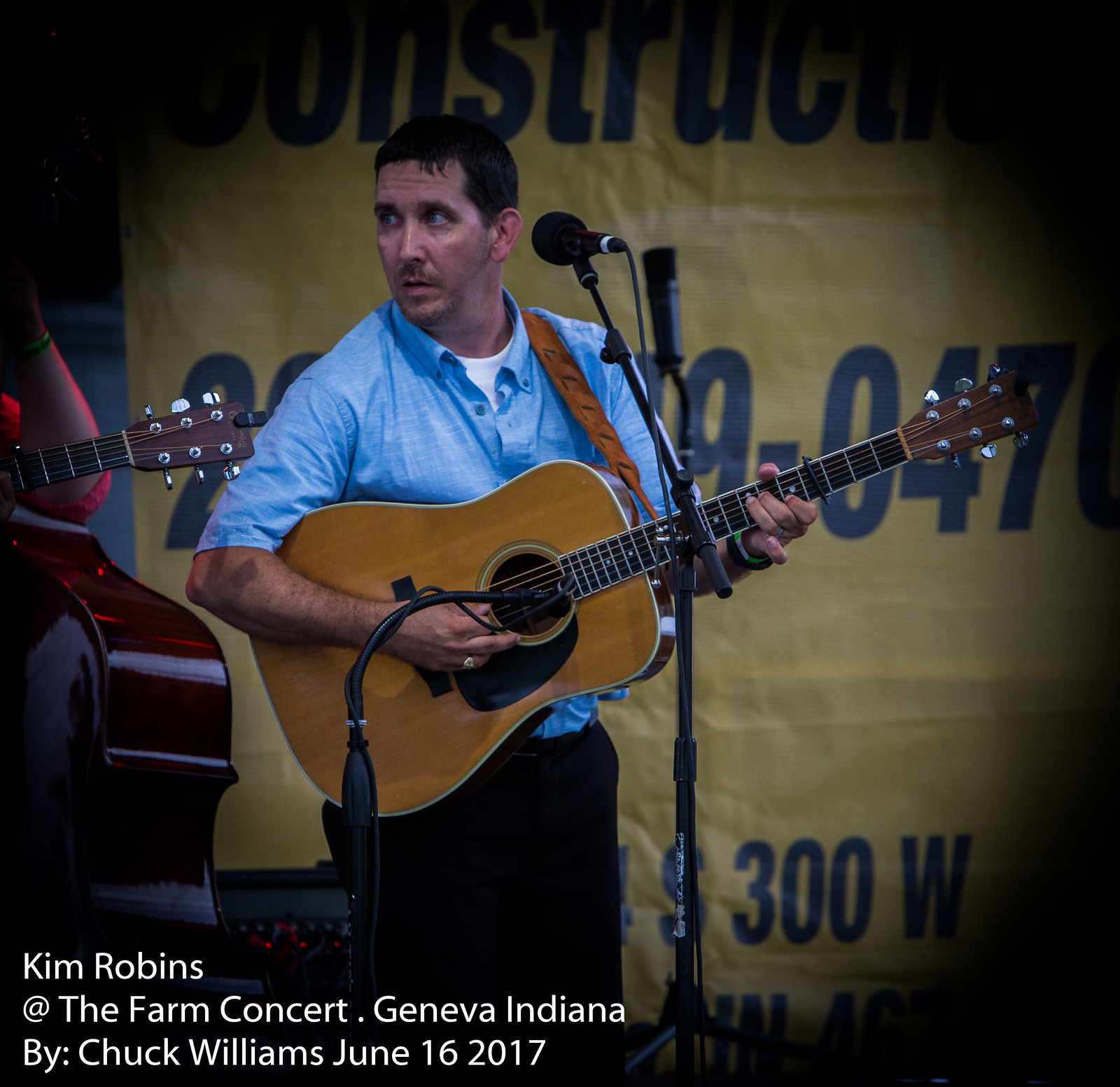In this image from the Farm Concert in Geneva, Indiana, taken by Chuck Williams on June 16, 2017, we see two musicians prominently featured. The main subject, Kim Robbins, is standing in the foreground, playing an acoustic guitar with a red strap. He is dressed in a short-sleeved blue button-down shirt over a white undershirt and sports black hair and a slight mustache. Kim is positioned in front of a black microphone, facing to the viewer's left but turned to the right from his own perspective. 

Behind Kim, there is another musician only partially visible. This second musician is playing an upright bass, as evidenced by the elbow resting on the instrument and part of the bass itself. The background of the image features a yellow sign with blue text, partially obscured by shadows around the picture edges. The text in the bottom left corner of the image reads "Kim Robbins at the Farm Concert, Geneva, Indiana by Chuck Williams, June 16, 2017," in white font.